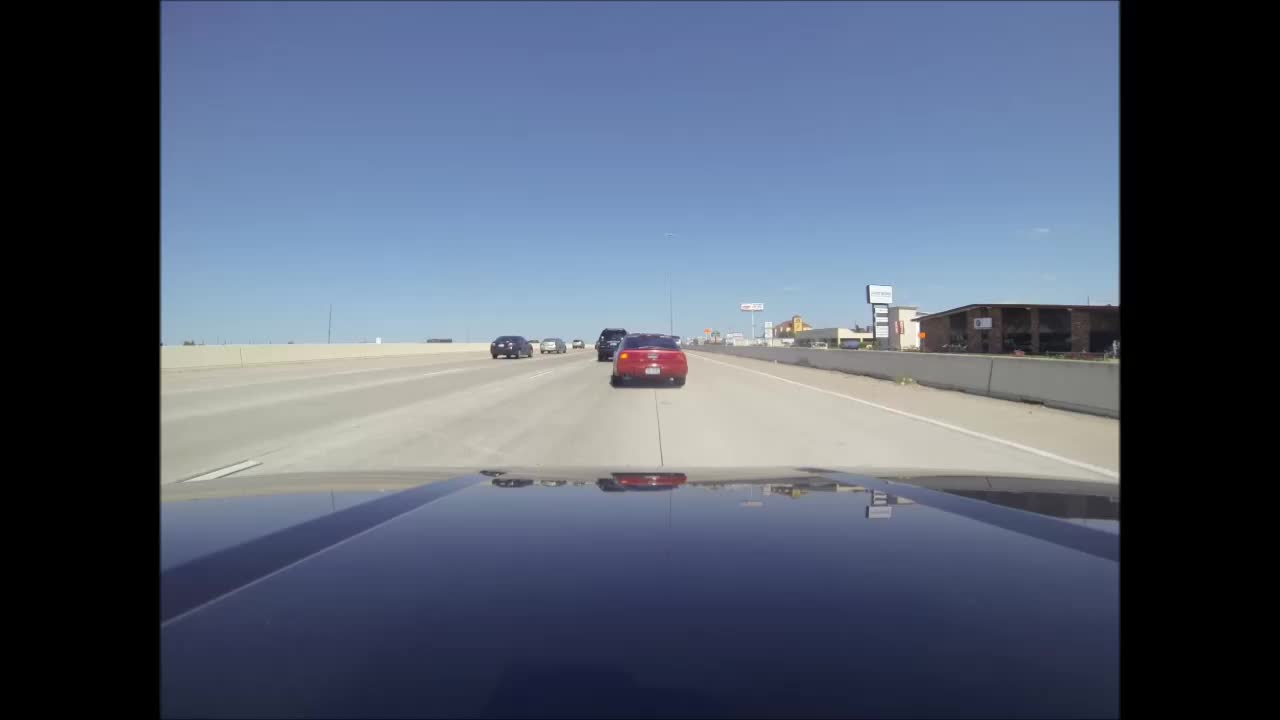This photograph, taken from a dash camera, captures the view of a black-hooded car driving on a three-lane highway. In the center lane, directly ahead, a small red sedan with black tinted windows and a white license plate is changing lanes with its left turn signal blinking. Additional cars are visible: a dark-colored SUV ahead of the red sedan and a dark blue sedan to the left. 

Concrete barriers line both sides of the highway. On the right-hand side, beyond the barrier, you can see multiple buildings and signs, consistent with urban roadside structures like car dealerships. A standout feature is a tall sign in the distance with a large white banner at the top and smaller banners descending along a black rectangle. There’s also a beige structure, possibly another sign, followed by a brick building with a reddish-brown facade and a dark brown trim. This building has a white rectangular sign with a small brown symbol to the left. The sky above is completely clear and vivid blue, contributing to the bright and sharply detailed scene.